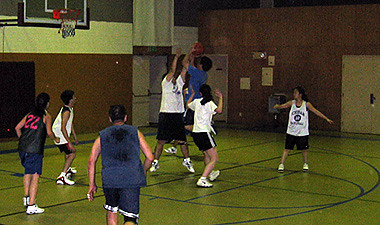In this vibrant indoor photograph captured within a gymnasium, a group of youthful basketball players, both male and female, are engaged in an intense game. The players are divided into two teams distinguished by their jerseys: one team in blue sleeveless shirts and the other in white t-shirts paired with dark shorts. The focal point of the image features two players in a dynamic standoff; one in a white t-shirt is defensively blocking the opposing player, who, clad in blue, is poised with the basketball, aiming to make a shot at the hoop which is positioned to the left. The basketball hoop juts out from the wall, featuring a clear backboard and a vibrant net in red, white, and blue. The court's floor is a distinctive greenish-gold hue, framed by brown walls that are accented with a gray stripe and a white stripe towards the top. Several doors are visible along the gym walls, and the lines marking the basketball court are clearly delineated. All players sport white sneakers and appear to be in the mid-teens, suggesting they are likely high school or eighth-grade students.